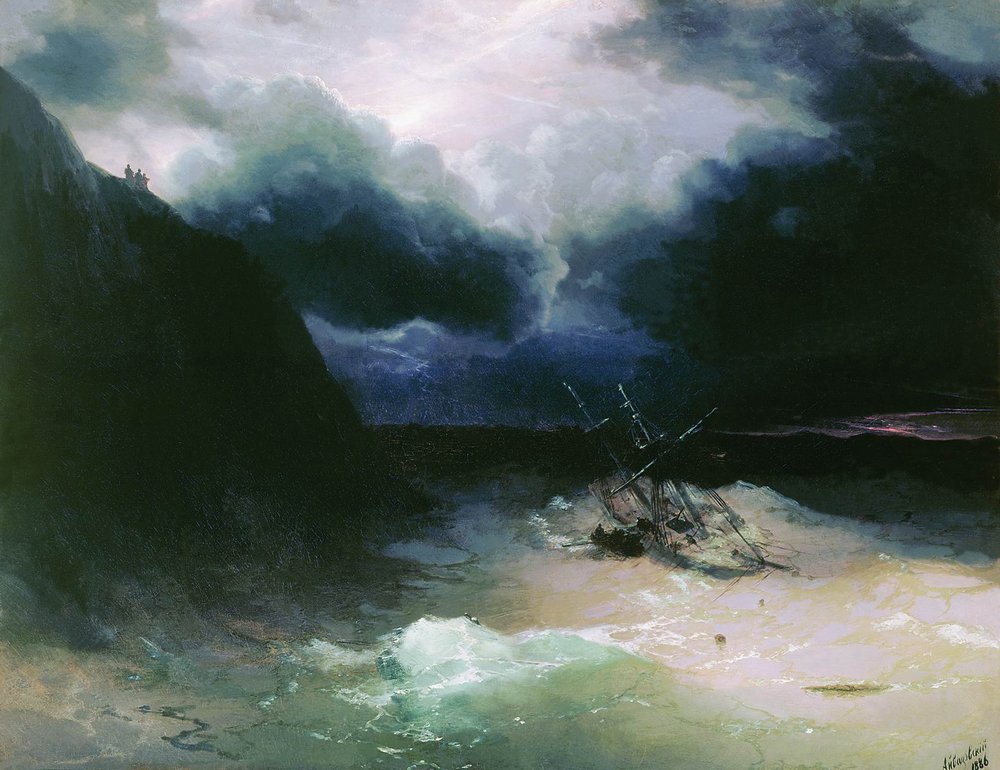The image is a detailed painting of a dramatic shoreline scene. The composition is horizontal and rectangular, capturing the tumultuous interaction between land and sea. The foreground features a sandy shoreline strewn with debris, including a large tree branch or possibly a whole tree that has been swept ashore by the waves. The water looks rough, with brown and greenish hues and white-capped waves crashing towards the shore, indicating a stormy sea.

Towards the center of the painting, a stranded boat appears to be wrecked on a small piece of land, hinting at a maritime disaster. The boat is being pummeled by the rough seas, adding to the scene's sense of turmoil and tension. The water's color and texture are well-rendered, highlighting the artist's skill, and the painting is marked with a signature in the bottom right corner, confirming its status as a hand-crafted work of art.

In the background, the landscape darkens, featuring either hills or cliffs. On the left side, a significant cliffside rises, where three tiny figures are barely visible, standing at the top and seemingly observing the chaotic scene below. The sky above is equally dramatic, filled with dark, angry clouds mingling with lighter ones, creating a moody and foreboding atmosphere.

Overall, the painting masterfully conveys a sense of nature's power and the cling of humanity amidst the storm.